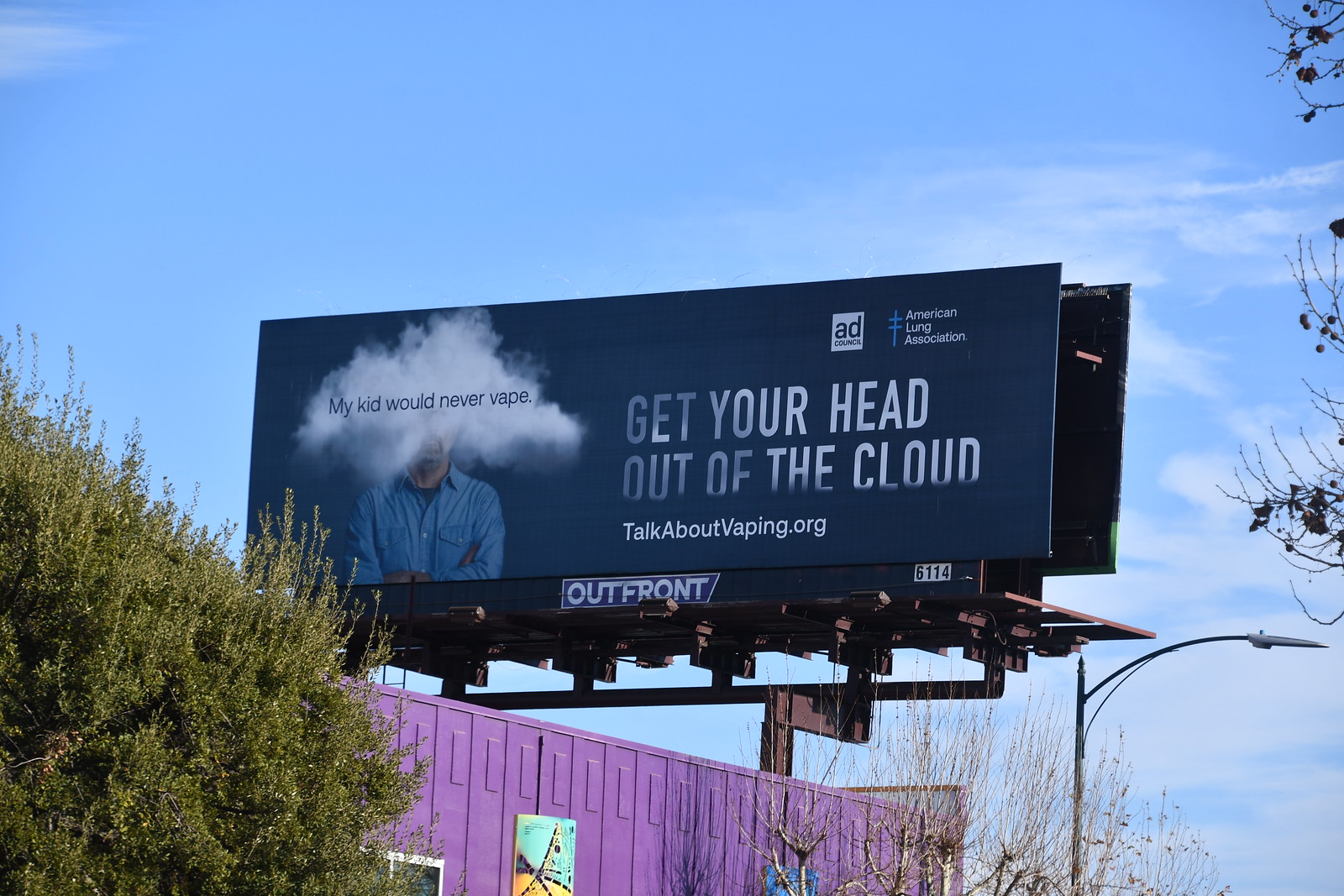The image depicts a highly realistic photograph of a large billboard. The billboard features an illustration of a parent with their face obscured by a cloud, accompanied by the text, "My kid would never vape." The parent, dressed in a light blue denim button-down shirt, is positioned centrally on the billboard. Beside the cloud, bold text reads, "Get your head out of the cloud," and below it, smaller text directs viewers to "talkaboutvaping.org." Above this text, the initials "AD" can be seen, suggesting the ad's production credentials. The American Lung Association is identified as the producer, indicating the advertisement's purpose to discourage vaping, targeting both kids and the general public.

Beneath the billboard, a purple wall adorned with various artworks is visible, adding an artistic flair to the urban setting. To the right of the wall stands a tree barren of leaves, while to the left, a tree with lush, green foliage contrasts starkly. The sky overhead is a vibrant blue, dotted with white, fluffy clouds, adding to the bright and airy ambiance of the scene.